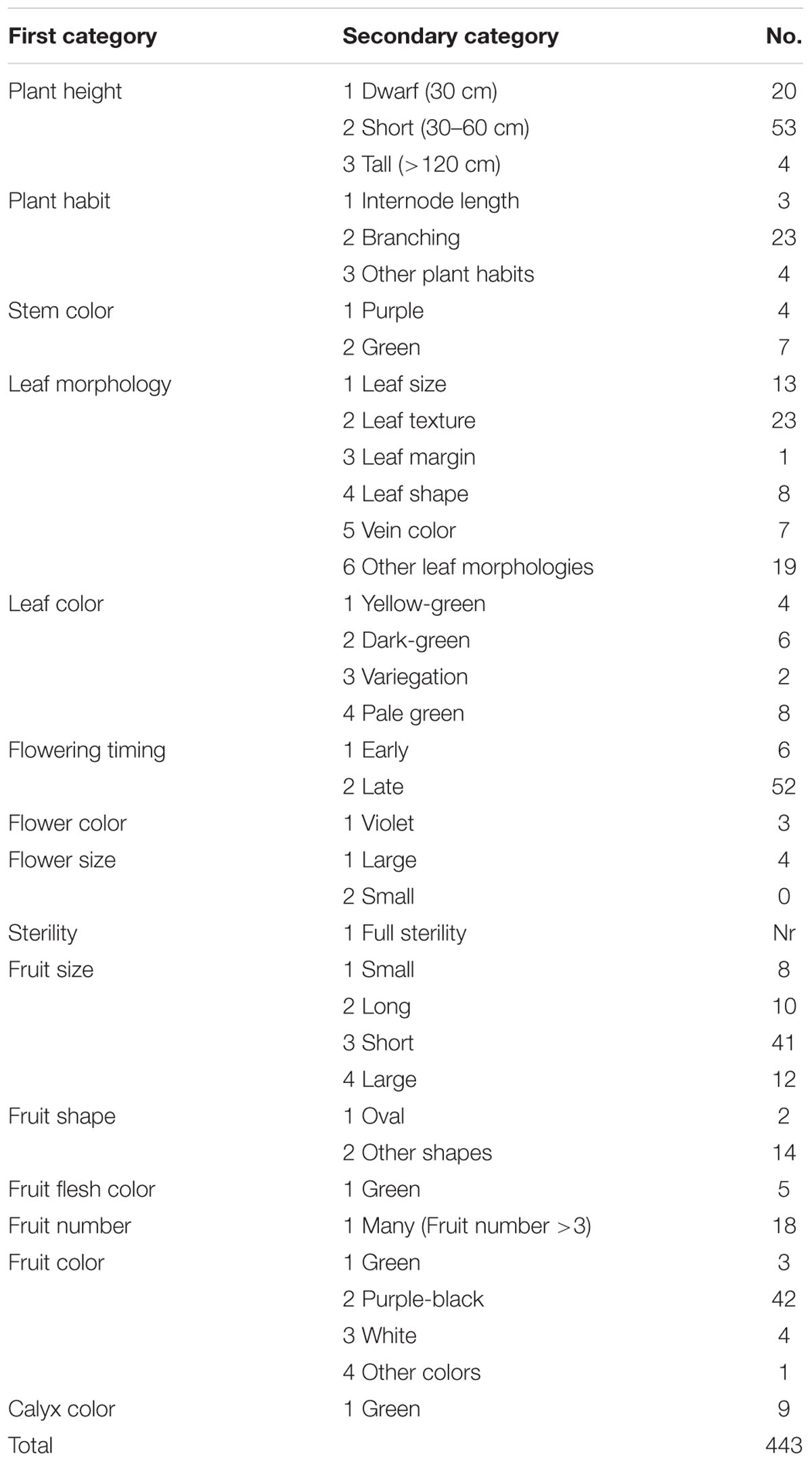This image is a screenshot of a detailed list against a white background with black font. At the top, there is a labeled rectangle categorizing data into two main sections: "First Category," "Second Category," and "No.," indicating a numerical section.

Under "First Category," the data is organized into various botanical attributes including:
- Plant Height
- Plant Habit
- Stem Color
- Leaf Morphology
- Leaf Color
- Flowering Timing
- Flower Color
- Flower Size
- Sterility
- Fruit Size
- Fruit Shape
- Fruit Flesh Color
- Fruit Number
- Fruit Color
- Calyx Color
- Total

Under "Second Category," more specific descriptors are listed with numerical indications such as:
- 1. Dwarf (30 cm)
- 2. Short (30-60 cm)
- 3. Tall (120 cm)
- 1. Internode Length
- 2. Branching
- 3. Other Plant Habits
- 1. Purple
- 2. Green
- 1. Leaf Size
- 2. Leaf Texture
- 3. Leaf Margin
- 4. Leaf Shape
- 5. Vein Color
- 6. Other Leaf Morphologies
- 1. Yellow Green
- 2. Dark Green

The categories and descriptors are meticulously listed to catalog the characteristics and measurements of different plants.